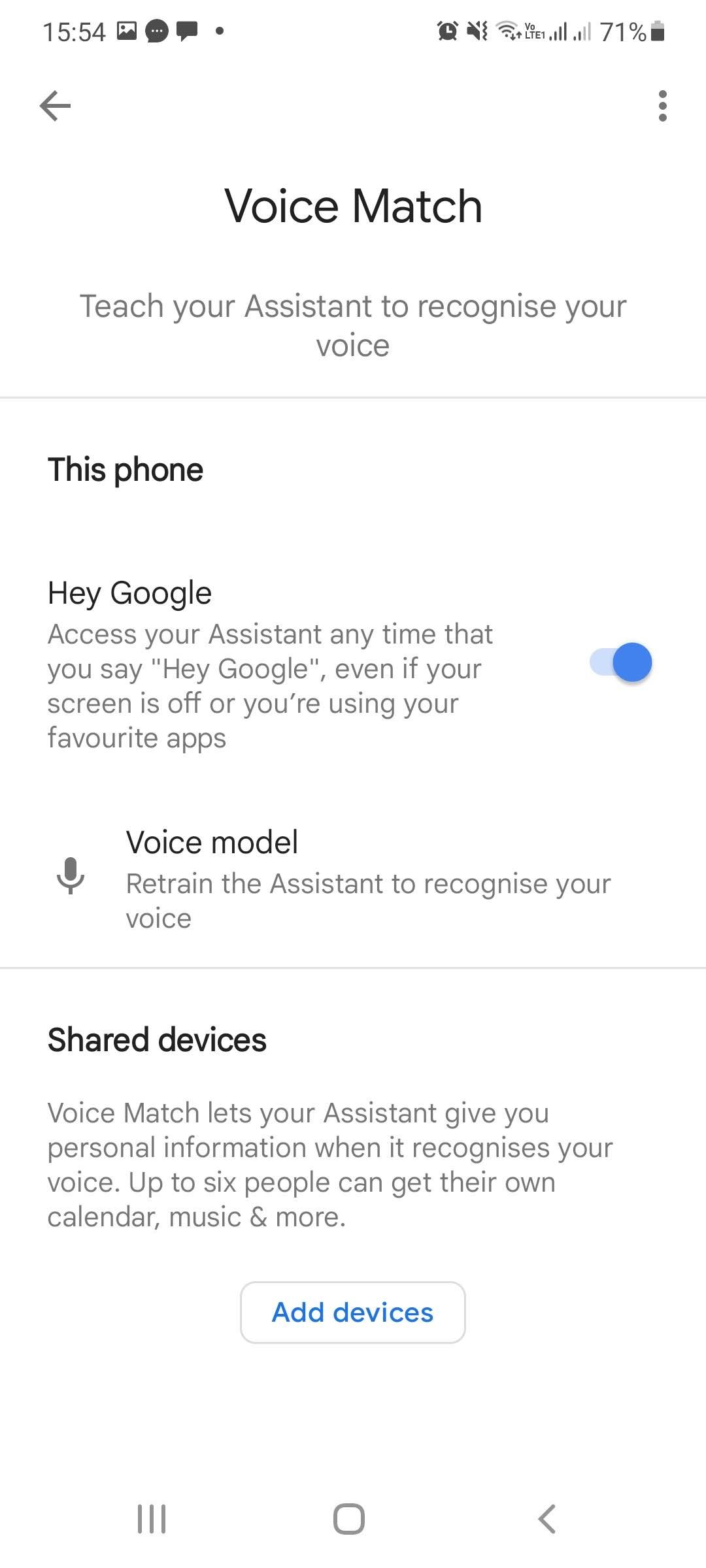This image captures a screenshot of a voice assistant application on a smartphone. The screenshot is in portrait orientation with a white background, lacking defined borders but maintaining typical cell phone proportions.

At the top of the screenshot, the status bar displays various icons against the white background. These include:

- The time "15:54" in black font.
- An image icon.
- Two distinct text message bubble icons.
- A dot indicating additional notifications.
- An alarm clock icon.
- Icons for silent and vibrate modes.
- A Wi-Fi connection symbol.
- Network signal bars.
- A percentage bar.
- A battery icon showing 71% charge.
- Another battery icon with a vertical black meter.

Beneath the status bar is a navigation bar featuring a black left arrow for going back and a vertically stacked three-dot menu icon.

The main section of the screenshot features a header titled "Voice Match," followed by the text, "Teach your Assistant to recognize your voice." A thin gray border separates this header from the following section titled "This Phone." This section includes:

- Instructions that say, "Hey Google, access your Assistant any time you say 'Hey Google,' even if your screen is off or you're using your favorite apps."
- A blue toggle switch indicating the feature is enabled.
- An option labeled "Voice Model," which allows you to retrain the Assistant to recognize your voice.

Below this is another section titled "Shared Devices," accompanied by a paragraph of additional information, and a gray box labeled "Add Devices" in blue font.

This detailed screenshot exemplifies the setup and options available within the voice assistant feature on the smartphone.